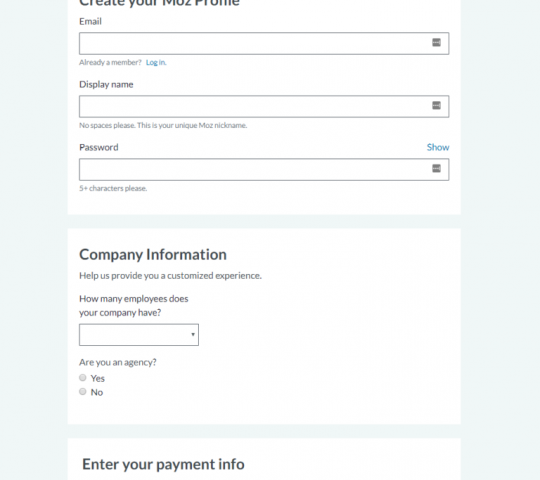A square-shaped image showcases a user signup page, possibly for a service named "Moz Phone." The top of the page features a partially visible title, likely reading "Create Your Moz Phone." Beneath the title, there are slightly cut-off instructions. The layout is organized into distinct sections, each clearly divided by light blue borders.

The first section is designated for email entry, featuring a rectangular text field. Below the email section is a display name field followed by a password field. This section is separated by a light blue divider from the next part, which is for company information entry. Another divider below the company section leads into the payment information section, although the details here are cut off within the image.

The main headings, such as "Create Your Moz Phone," "Company Information," and "Enter Your Payment Info," are prominently bolded for clarity. The form fields, each rectangle-shaped, facilitate structured information entry. The page layout ensures an orderly and user-friendly sign-up process, highlighted by the clear segmentation and distinct borders.